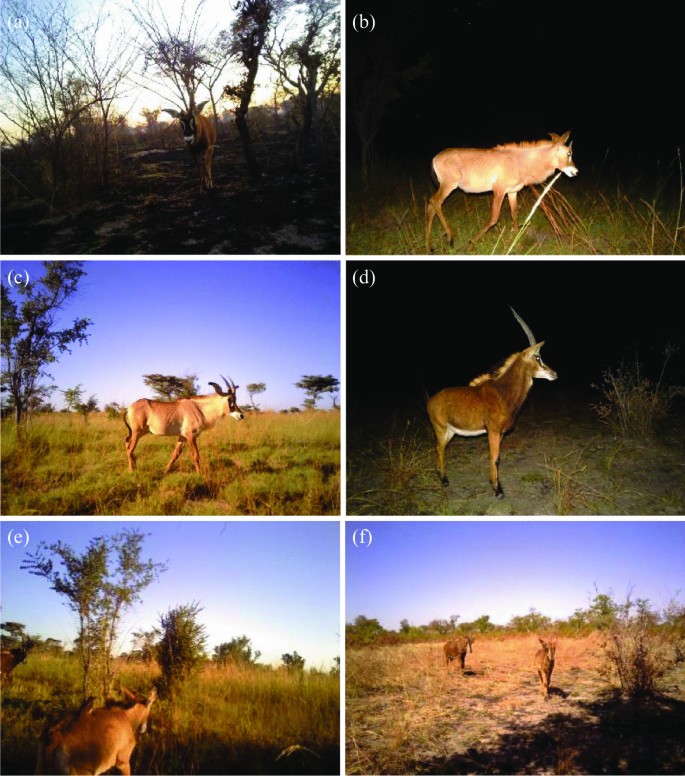The image is a collage of six outdoor wildlife scenes labeled A through F, featuring animals in various natural settings. Image A, in the top left, shows a goat in a sparse fall or winter forest with bare trees and scattered leaves, captured under a partly cloudy sky with a darkened foreground. Image B, next to it, depicts a brown goat or ram at night, facing right, illuminated by a light source against a dark sky with a patch of visible grass. Image C, in the middle row, left side, features a ram during the day in a grassy field with sparse trees and a clear blue sky. Image D, beside it, shows another goat or ram with a long, straight horn, standing in the grass at night, also facing right. Image E, in the bottom left, presents a third-person view of a goat’s backside as it runs through a grassy field during the day, with more trees and a blue sky in the background. Finally, Image F, in the bottom right, captures two brown goats or donkeys walking towards the camera in a daytime grassy field, with sparse grass patches and green trees on the horizon.